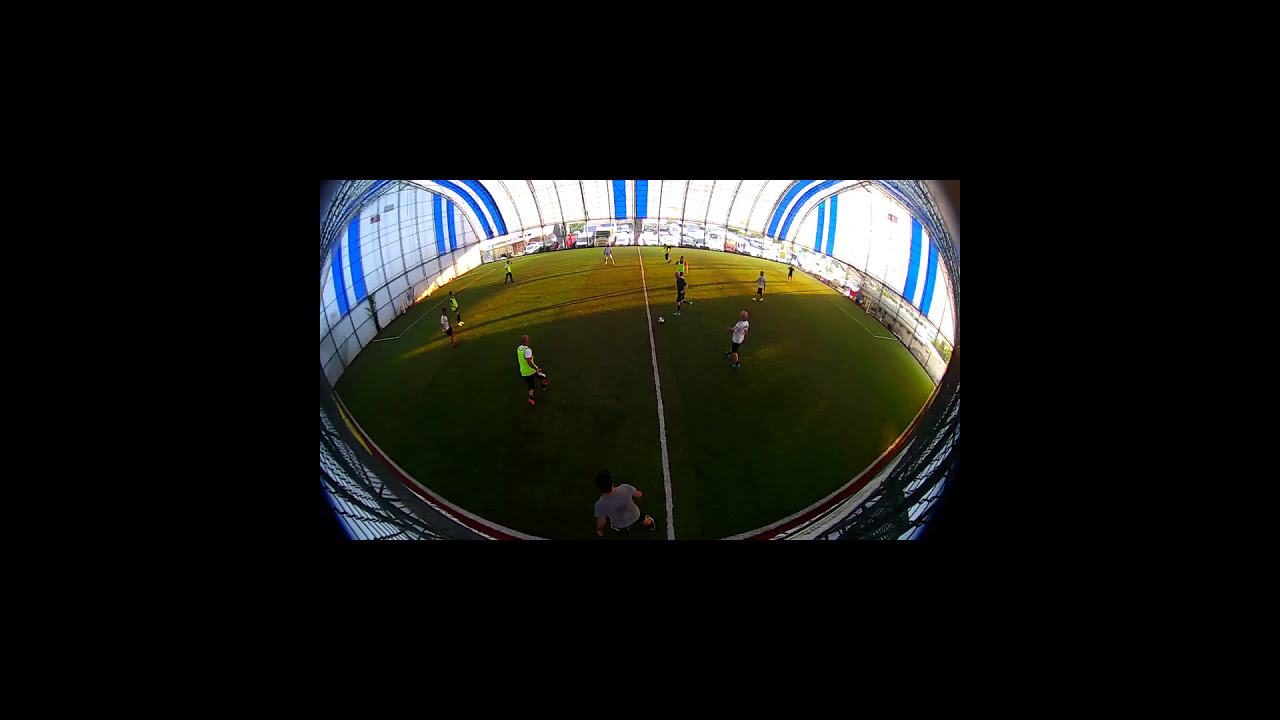The image depicts an indoor soccer stadium with a fisheye lens perspective, creating a warped effect that makes the walls appear to curve in and out. Dominating the scene is a centrally positioned grassy field, marked with white paint lines, possibly natural or artificial turf. The field is populated with numerous players, including a referee overseeing the game. Surrounding the field is a massive black border that takes up a significant portion of the image, amplifying the enclosed atmosphere. The stadium itself is notable for its circular design, accentuated by stained glass walls that allow sunlight to flood in, suggesting it might be late in the evening. The overall color palette includes black, various shades of green, blue, white, gray, and tan. In the background, there are visible vehicles, hinting at a parking lot outside, further illuminated by the sunlight streaming through the stained glass.